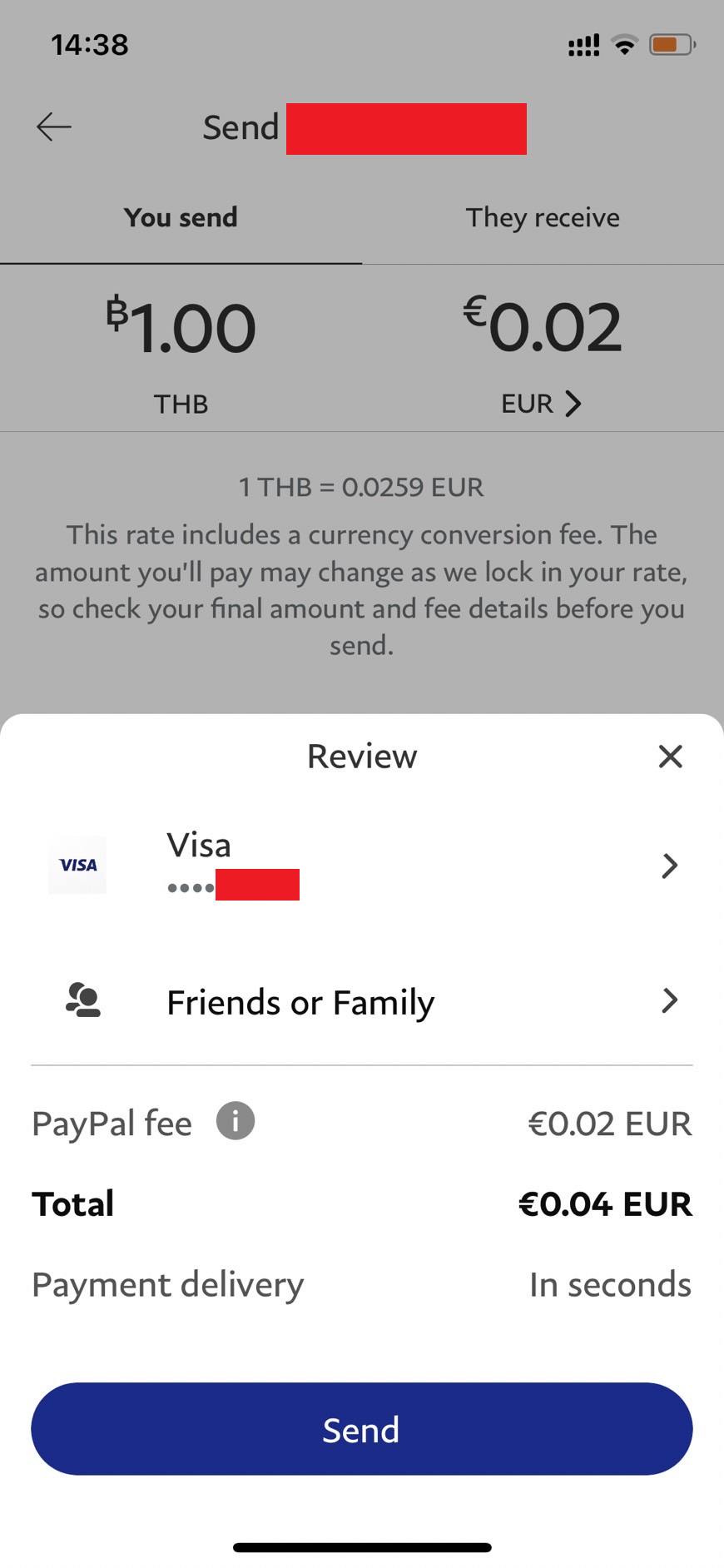In this screenshot of a PayPal transaction page, the interface is easily recognizable with its characteristic design elements, such as the font, buttons, and overall language design style. The image is divided into two distinct sections: a slightly blurred background and a more prominently focused review section.

In the dimmed background, the initial screen for sending money is visible. It clearly states "Send Money" at the top, and the transaction involves the Thai currency, abbreviated as THB. Specifically, the amount being sent is 1 THB, which is equivalent to 0.02 euros.

The foreground is the review section, which stands out with a sharper white background. Here, the specifics of the transaction are detailed. The money is being sent from a Visa card, likely a quick check due to the trivial amount involved. Notably, a PayPal fee of 0.02 euros is applied to this transaction, thereby doubling the total to 0.04 euros. At the bottom of the review section, it reassuringly states that payment delivery will occur in seconds.